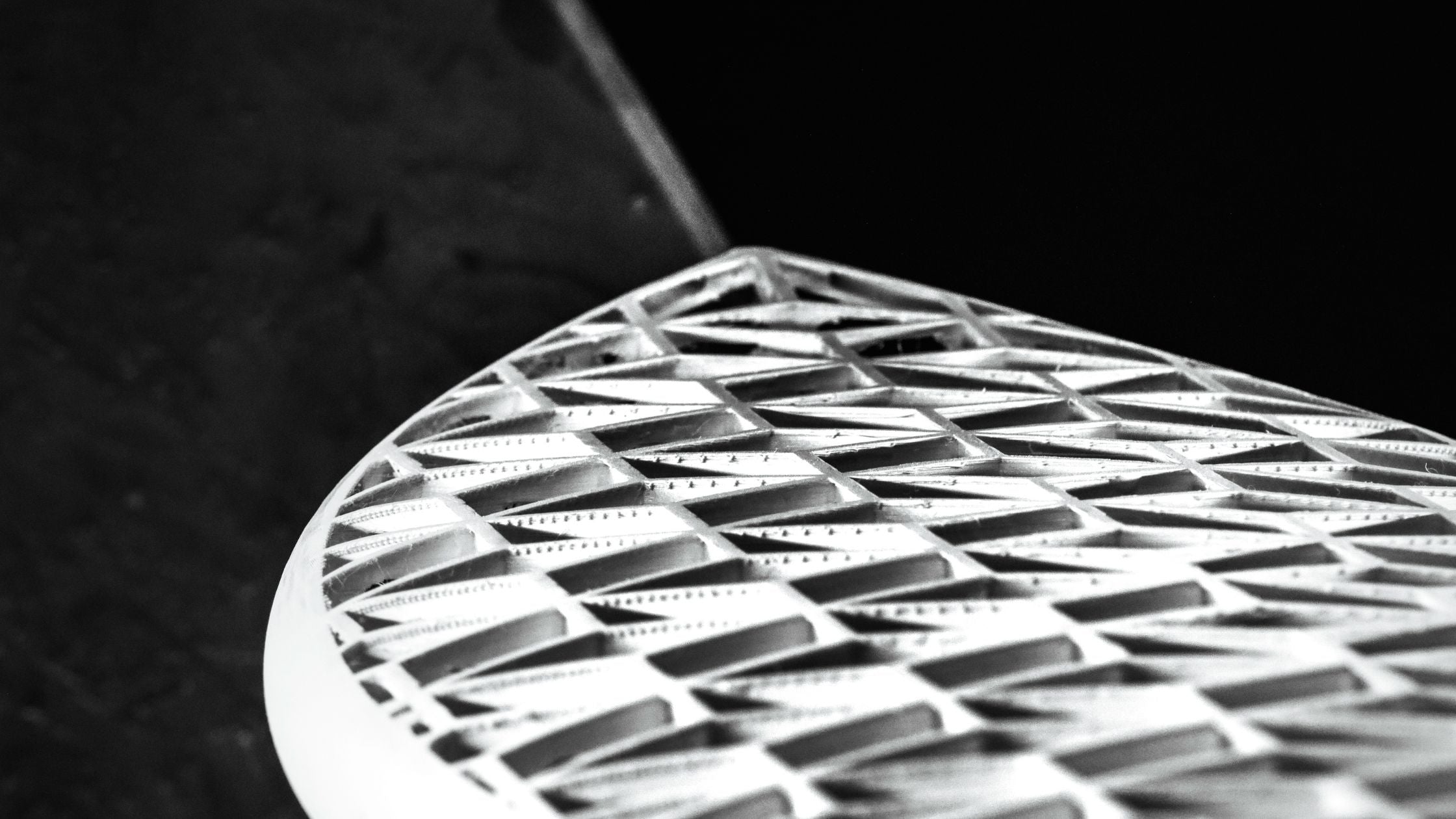The image is a highly magnified, black-and-white close-up of a metallic object set against a predominantly black background. The object begins in the lower right-hand corner and extends upward to the left, occupying two-thirds of the space. It is shaped somewhat like a leaf or a canoe, ending in a pointed tip. Emerging from this point is a light gray stick or line that extends vertically through the black background. The surface of the object is irregular, featuring distinct, indented square patterns. Each square houses two triangles pointing upwards to the left, with the central squares clearly showing small black dots within the triangles. The outer squares are less discernible due to the lighting. The texture of the object is very detailed, with raised parts and tiny points, making it resemble a futuristic or mechanically intricate item, possibly a space station or a tool under magnification. The photograph's close-up nature makes it difficult to identify the object definitively.